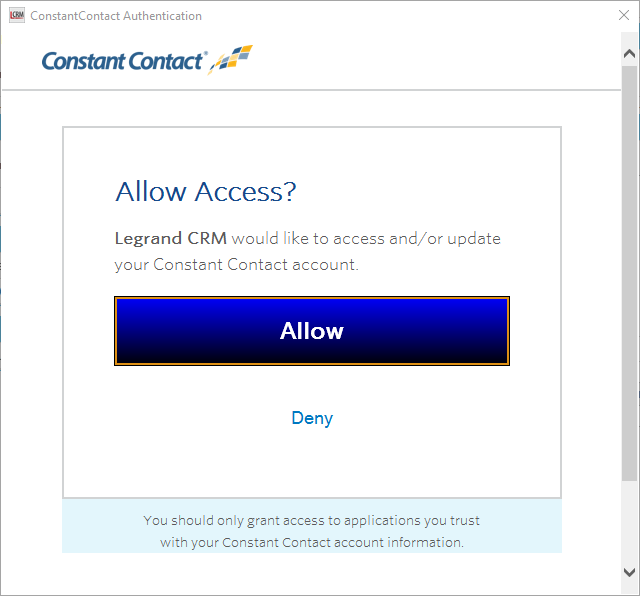The image depicts a website interface from the company Constant Contact Authentication, displayed on a computer screen. The website features a predominantly white background with the company's logo prominently displayed. The logo includes the text "Constant Contact" in a combination of orange, brown, and black colors, accompanied by a wavy flag-like symbol composed of blue, gold, and white boxes. 

On the right-hand side, there is a gray slider bar. Centered on this white background, a pop-up window appears with the message in blue text: "Allow access?" Below this, in black text, it states, "Lagrand CRM would like to access and/or update your Constant Contact account." The pop-up features a prominent blue button outlined in orange, with the word "Allow" written in white. Below this button, against the white background, there is a light blue "Deny" option.

At the bottom of the pop-up, a blue box contains a cautionary message advising users: "You should only grant access to applications you trust with your Constant Contact account information."